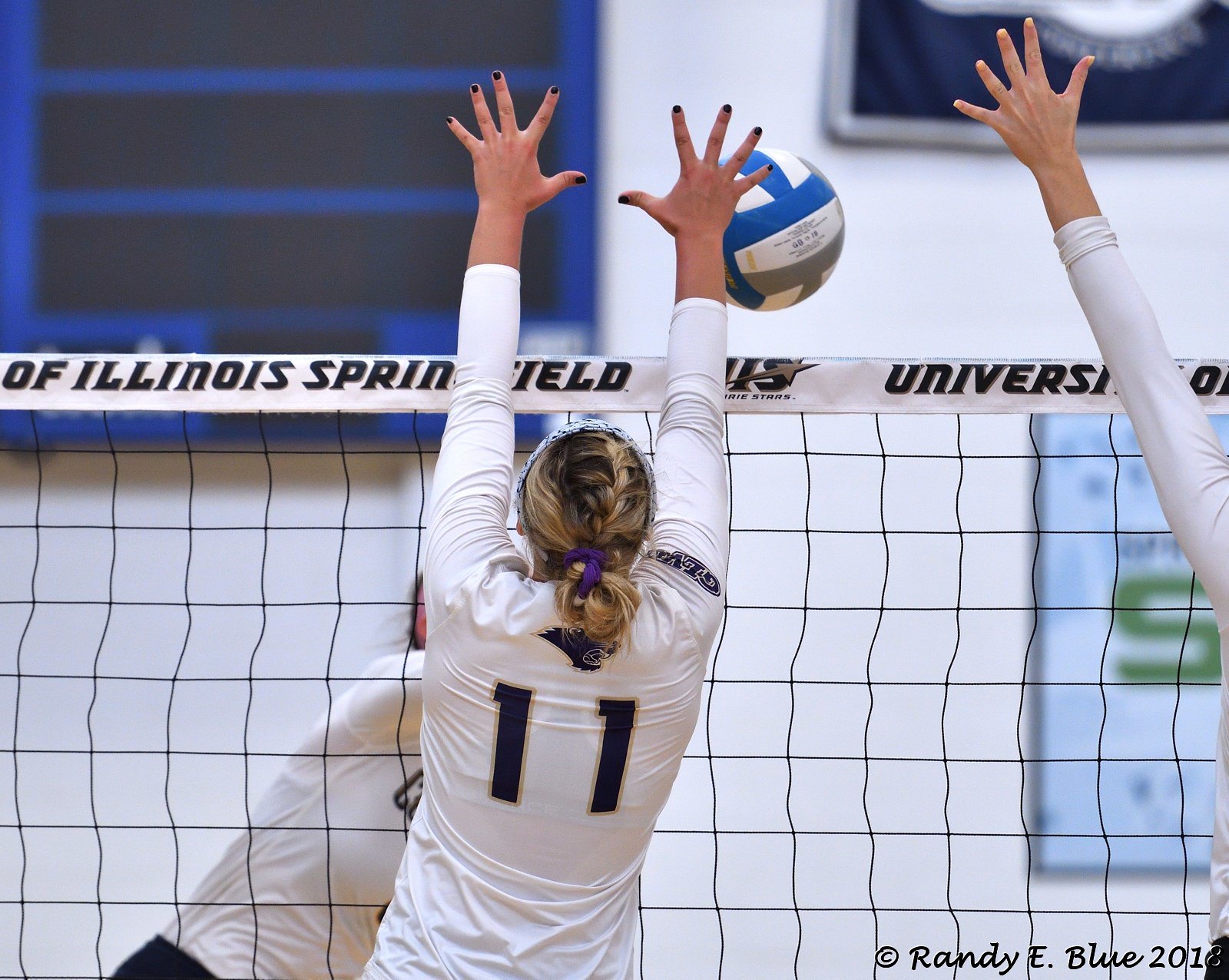The image depicts an intense moment during a university women's volleyball match, likely taking place inside a gymnasium. Prominently visible is a player from the University of Illinois Springfield team, wearing a white long-sleeve jersey numbered 11. She has blonde hair styled in a ponytail with a purple scrunchie, complemented by a headband, and her nails are painted black. The player is captured mid-jump, with both hands raised in an attempt to block a multi-colored volleyball (white, gray, and blue) flying over the net. The net, which has white piping and black strings, stretches across the image from left to right. Above the net, the words "University of Illinois Springfield" are discernible. A watermark in the bottom right corner indicates "Copyright Randy E. Blue 2018." The court is flanked by a blank scoreboard in the top left corner and various banners, including one with a green "S" and another partially visible on the top right. Only one of the three players on the volleyball team is fully visible, with the arm of another player attempting to block the ball appearing on the right side of the image. The background features a white wall and additional banners with black rectangular elements.